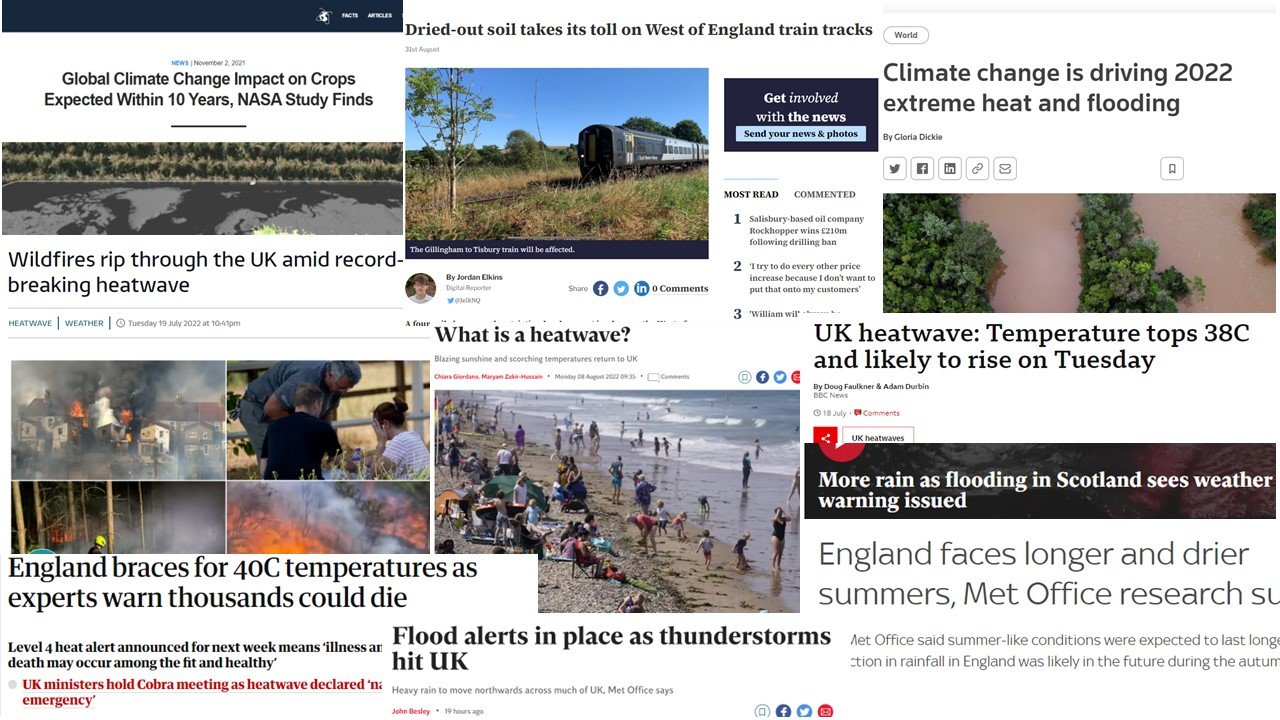A comprehensive emergency news webpage dated Monday, August 8, 2022, at 9.35 AM reports on a series of alarming events and studies related to climate change impacts in the UK. Key headlines include a NASA study predicting significant impacts on crop yields due to climate change within the next decade, and reports of dried-out soil severely affecting train tracks in the West of England. The page also highlights the destructive wildfires currently spreading across the UK as a result of an unprecedented heatwave. Amidst record-breaking temperatures, England is preparing for a staggering 40 degrees Celsius, with experts warning that thousands could succumb to the extreme heat. A Level 4 heat alert, the highest possible, has been announced for the upcoming week, indicating that serious illness and death may occur even among healthy individuals. In response, UK ministers have convened a Cobra meeting as the heat wave has reached the level of a national emergency. Additionally, the page offers an explanation of what constitutes a heat wave, as blazing sunshine and soaring temperatures continue to impact the UK. Flood alerts have also been issued following a bout of thunderstorms, and new research from the Met Office suggests that England is likely to experience increasingly longer and drier summers.